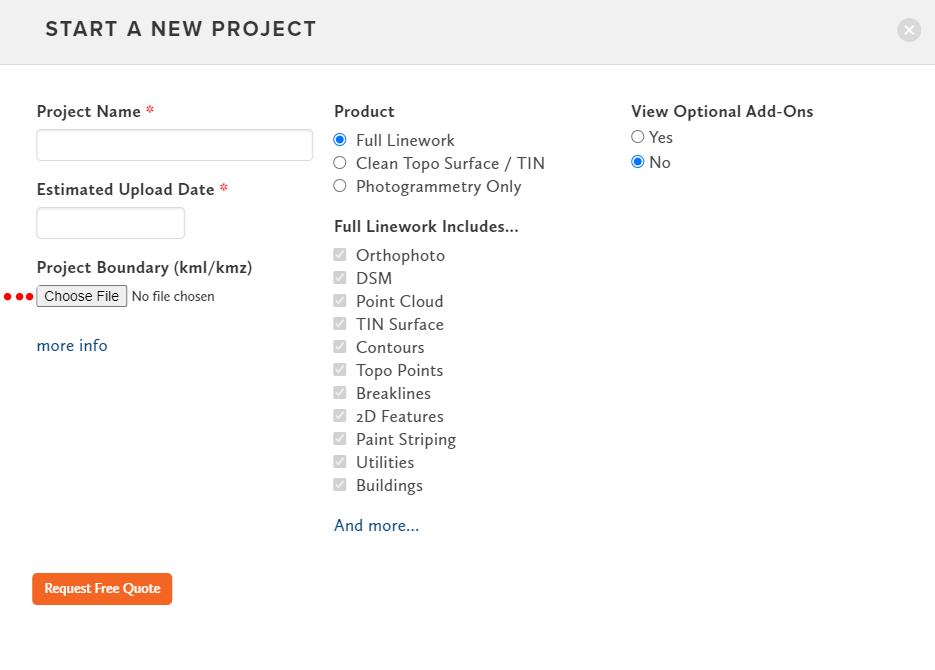The image is a screenshot from a website or app, presented in a landscape orientation. At the very top is a gray rectangle labeled "Start a New Project," with an "X" button on the far right for closing this option. Below it is a white box labeled "Project Name" marked with a red asterisk, indicating a required field where users can type in the name of their project. 

Further down is another field labeled "Estimated Upload Date," also marked with a red asterisk, followed by a text box for user input. The section continues with a label "Project Boundary KML/KMZ" next to a button labeled "Choose File," accompanied by three red dots. Currently, no file has been chosen. Below this is a link labeled "More Info" for additional details.

On the left-hand side of the image, there is an orange button labeled "Request Free Quote." Moving to the middle section, there is a heading labeled "Product" with three radio buttons underneath. The options are: "Full Line Work," "Clean TOPO Surface/TIN," and "Photogrammetry Only." Presently, "Full Line Work" is selected, indicated by a blue dot in the center of the corresponding radio button.

Underneath the radio buttons is a list of items accompanied by grayed-out checkboxes, indicating they are not currently active. The items listed are: Orthophoto, DSM, Point Cloud, TIN Surface, Contours, TOPO Points (spelled out as T-O-P-O), Break Lines, 2D Features, Paint Striping, Utilities, Buildings, and more, which can be accessed via an additional link.

Finally, on the right-hand side, there is text that reads "View Optional Add-ons," with options to choose either "Yes" or "No." At the moment, "No" is selected.